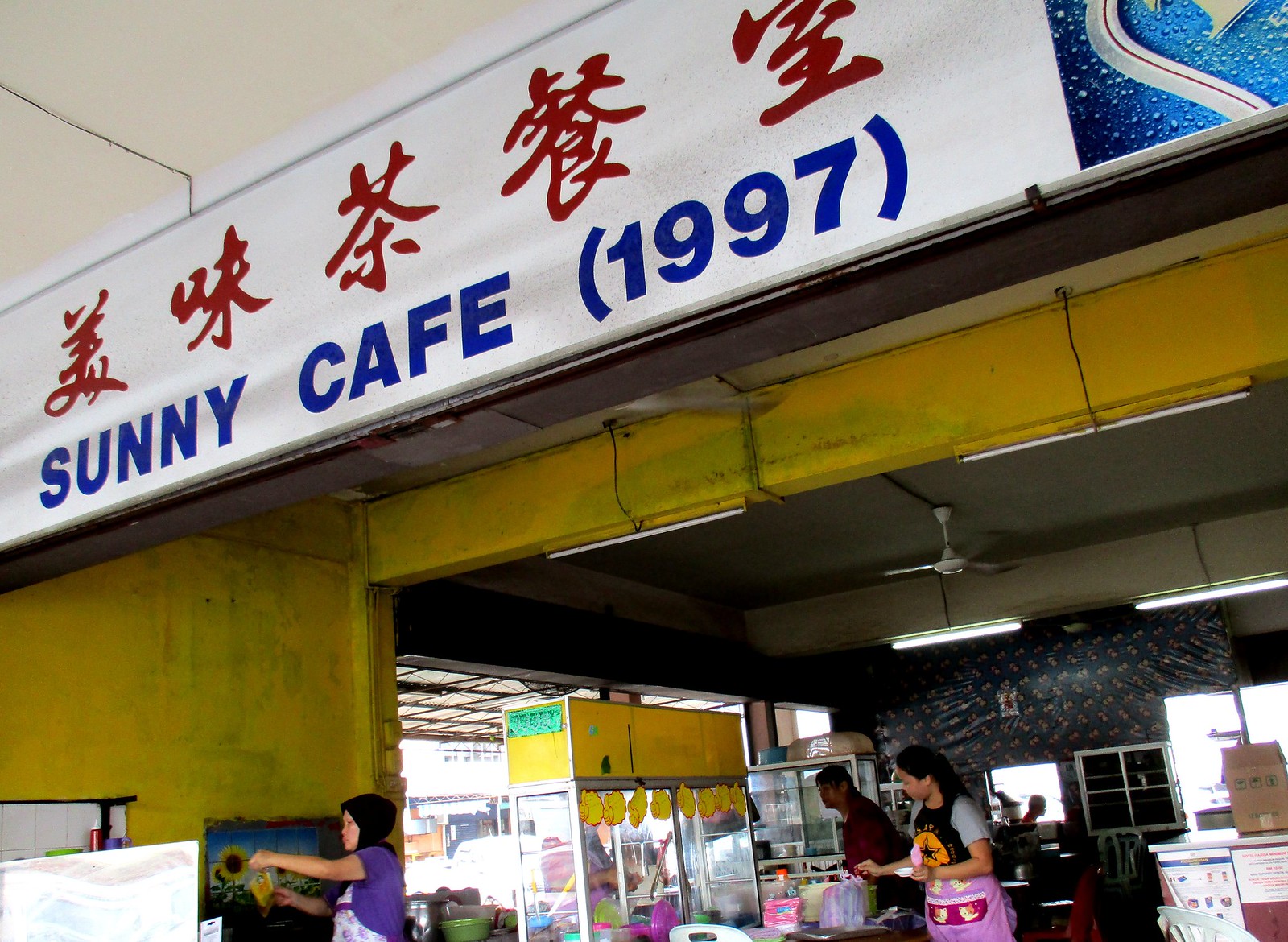The photograph captures a yellow-walled cafe storefront, whose paint is peeling to reveal hints of green beneath. A white banner, prominently displaying five red Asian characters above the blue text "Sunny Cafe, 1997," hangs above the large doorway. Inside, the scene is a bustling mix of activity; the shop is modest and slightly disheveled with plastic tables and chairs scattered about. 

In the center stands a yellow-topped plastic display case filled with jars and dishes, while a double-doored cooler at the back wall showcases an array of drinks. The ceiling fan spins overhead, adding to the quaint, old-world charm. Within this lively setting, three individuals are engaged in various tasks: a woman in a purple shirt and hijab pours something at the left, positioned in front of a sunflower painting; another woman in a gray t-shirt decorates a cake towards the lower center-right, and a person dressed in red observes from a distance. The photograph, taken indoors during the day, vividly conveys the unique atmosphere and character of the Sunny Cafe.